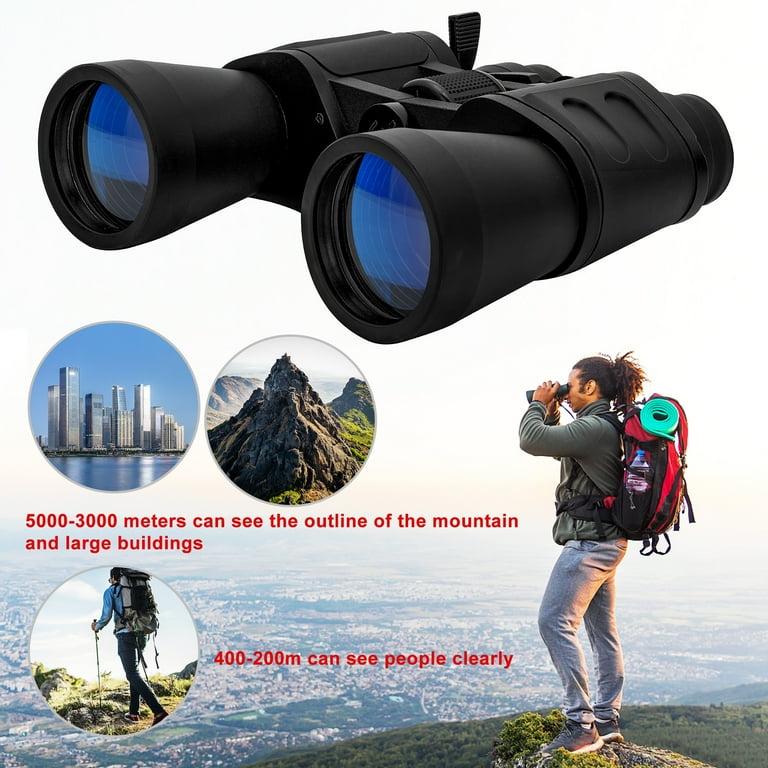The image is a square, 6 inches by 6 inches, featuring a detailed product photo of a pair of black binoculars with blue lenses against a white background in the top half. Below, a series of illustrative photographs demonstrate the use of these binoculars. In the center of the lower half, a man with black hair tied in a ponytail, brown skin, and wearing a long-sleeved gray shirt, gray pants, gray shoes, and a red and gray backpack, stands at the edge of a hill or cliff. He faces left with his arms raised, using the binoculars to look out over a distant city. To the left of him, two circular inset images showcase the binocular's capabilities: the left circle shows a city skyline and mountain peak with blue sky and water underneath, labeled with red print stating "5,000-3,000 meters can see the outline of the mountain and large buildings," and the right circle shows a hiker ascending a hill with red print stating "400-200 meters can see people clearly."